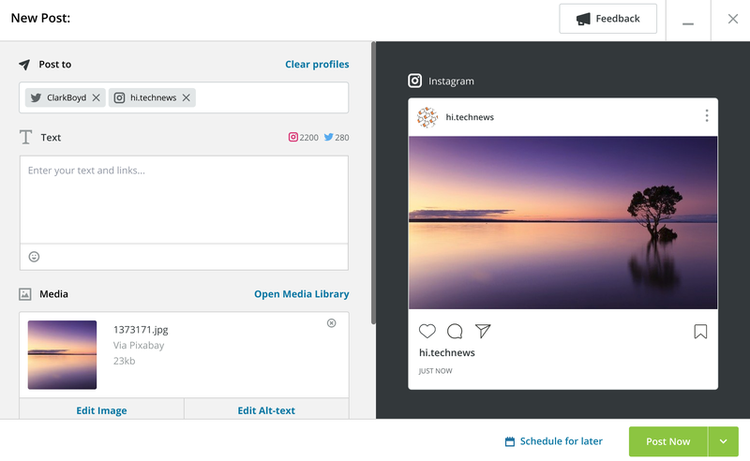"An Instagram post creation interface is displayed. In the upper left corner, the label 'New Post' is visible, indicating a new content upload. The upper right corner features several buttons including a megaphone icon labeled 'Feedback,' and options to minimize or close the window. Beneath these, the interface indicates the post will be shared across multiple platforms, listing 'Clark Boyd with an X on Twitter' and 'hi.technews on Instagram.'

A central text field, bordered by a large 'T' icon, is shown as blank and grey with the placeholder text 'Enter your text and links...'. It specifies that Instagram allows 2,200 characters and Twitter 280 characters, with these counters likely decreasing as text is entered. Alongside the text field, an emoji icon suggests that users can add emojis to their post.

Below this is a media section displaying a photo inset of a serene landscape with a tree growing out of a tranquil lake at sunset. This section is titled 'Media' and includes an icon of a mountain with the sun. Further options enable users to open their media library, and details such as the file name '1373171.jpeg' from Pixabay with 23K views are displayed. Additional buttons allow for editing the image or adding alt text.

On the right side of the interface, a preview shows how the post will appear on Instagram, featuring the profile icon of 'hi_technews,' a heart, a speech bubble, a share icon, and a bookmark icon, all accompanied by a 'Just Now' timestamp. At the bottom, users can choose to schedule the post for later with a calendar tool or instantly publish using the green 'Post Now' button in the bottom right corner."